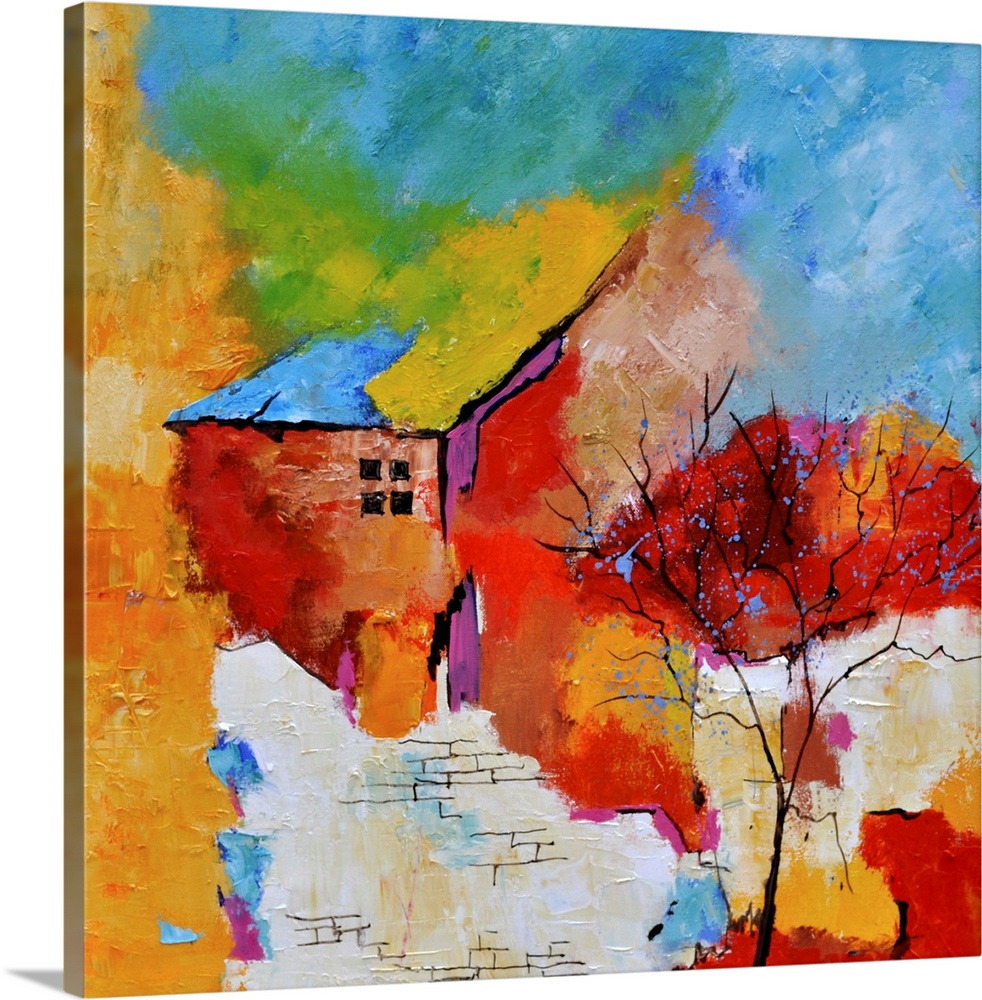The painting is a vibrant and abstract impressionist piece displayed on an upright canvas, with its slight shadow visible behind it. The focal point is a house or building distinguished by a blue roof and vividly painted walls - the left wall in striking red with four black-drawn square windows, and the right wall in a contrasting purple hue. Below this, the base of the building features a white brick wall or foundation.

In the foreground, a tall, slender black tree with thin branches stands in front of the building. The tree’s foliage is depicted in a dynamic blend of warm colors, including deep red, orange, pink, and yellow, appearing almost like colorful blobs.

The background is a lively burst of colors: a vertical orange rectangle occupies the left side from top to bottom, adjacent to a patch of green. To the right, the sky transitions into a bright blue, which stretches across the top half of the canvas, interspersed with blotches of orange, green, and yellow. The painting’s composition and exuberant palette create a vivid and beautiful effect, emphasizing its abstract, impressionist style.